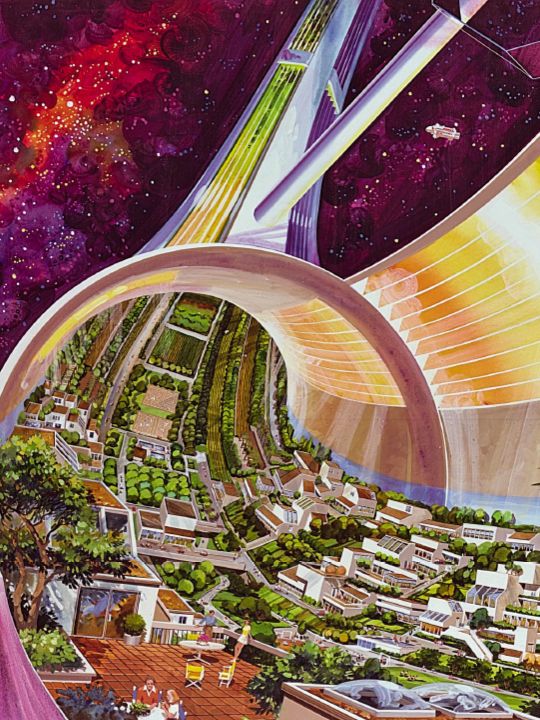This painting captures a vivid, futuristic vision of a space colony set within a large, curved capsule or ring that's suspended in the cosmos. The interior of this capsule, which features walls painted in shades of purple and yellow, resembles a self-sufficient community with a variety of elements intended to provide a semblance of Earthly life. The scene inside shows an abundance of greenery, including numerous plants and trees, suggesting agricultural efforts to sustain the inhabitants. Specks of white stars dot the purple and red expanse of the universe that surrounds the capsule. Additionally, the ring-like structure houses several typical California-style homes nestled among green bushes, demonstrating a domestic side to this space-bound society. There are also people visible inside the capsule, some standing and some seated, emphasizing the communal aspect. The top corners of the painting illustrate more of the external space environment, featuring a spaceship in the top right and a cloudy nebula in the top left. This highly detailed and nostalgic representation echoes the 1970s artistic notions of a futuristic civilization living in high-tech, self-contained habitats amidst the stars.